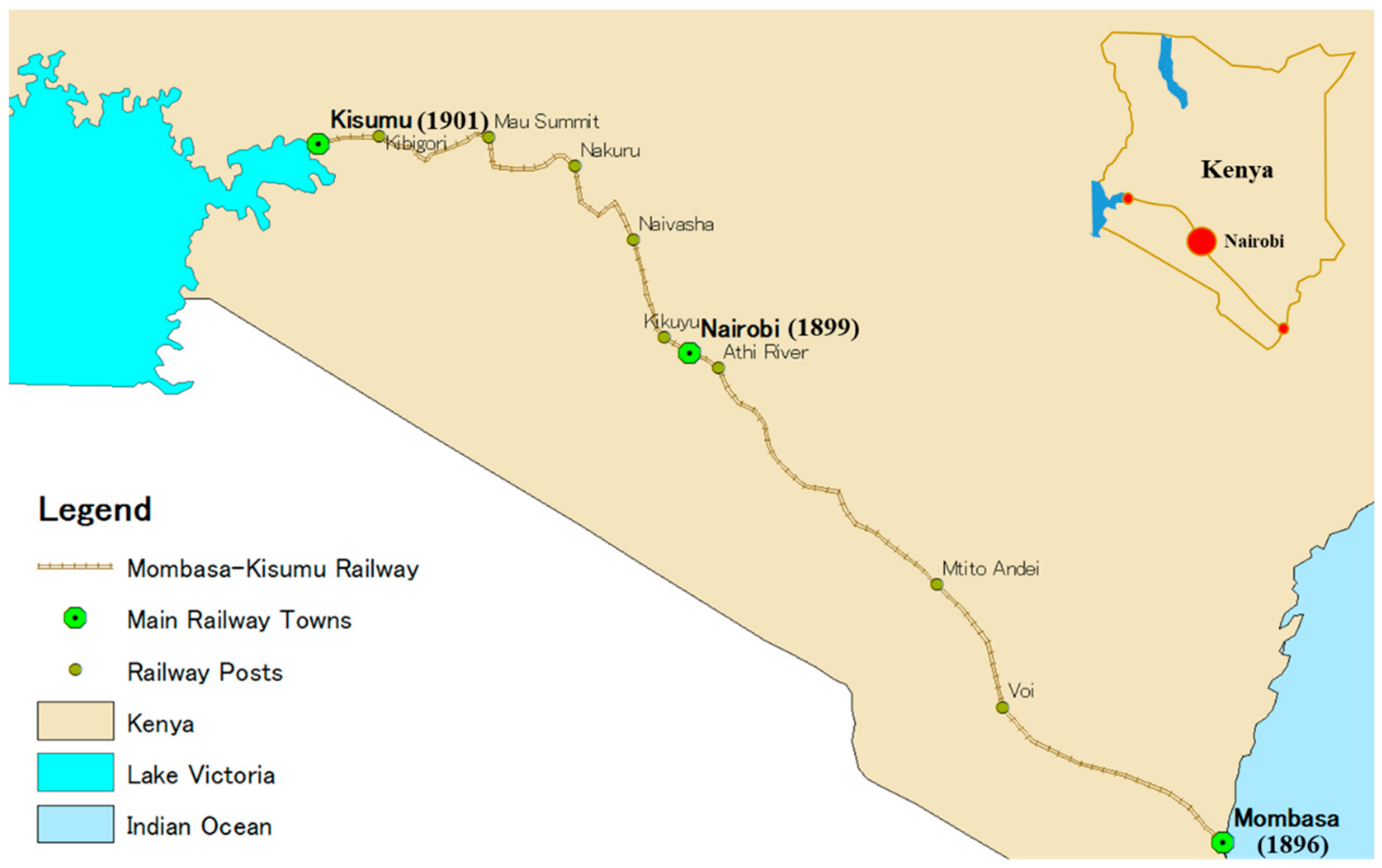This image features a detailed, colored map highlighting the southern region of Kenya. The main area of the map is predominantly pink, with a white portion in the bottom left containing a legend. The legend, titled "Legend," uses black text to describe various symbols. 

In the upper left, there is a bluish-green area mapped out, transitioning to a large pink area that dominates the map. The bottom right corner of this pink area is light blue, representing the Indian Ocean. Key locations along a railway line are marked with green circles; these include Mombasa (indicated by a green circle with a black dot and labeled “Mombasa” with “1896” in parentheses), Nairobi (similarly marked with “Nairobi” and “1899” in parentheses), and Kisumu (“Kisumu” with “1901” in parentheses). Additional towns and cities along the railway are also marked.

In the upper right corner, a small yellow outline delineates Kenya, with the region shown on the main map corresponding to the lower part of this outline. Nairobi is listed in the lower part of Kenya within this outline. The Kenyan region is depicted in light tan, and water bodies, including Lake Victoria in bright neon blue and the Indian Ocean in a light dull blue, are marked. 

A key within the legend indicates that the railway shown is the Mombasa-Kisumu railway. It distinguishes between the main railway towns (marked in bright neon green) and railway posts (marked in dull pea green). The map captures the geographic and infrastructural details of southern Kenya, providing a comprehensive overview of important cities and railway connections from the late 19th to early 20th century.